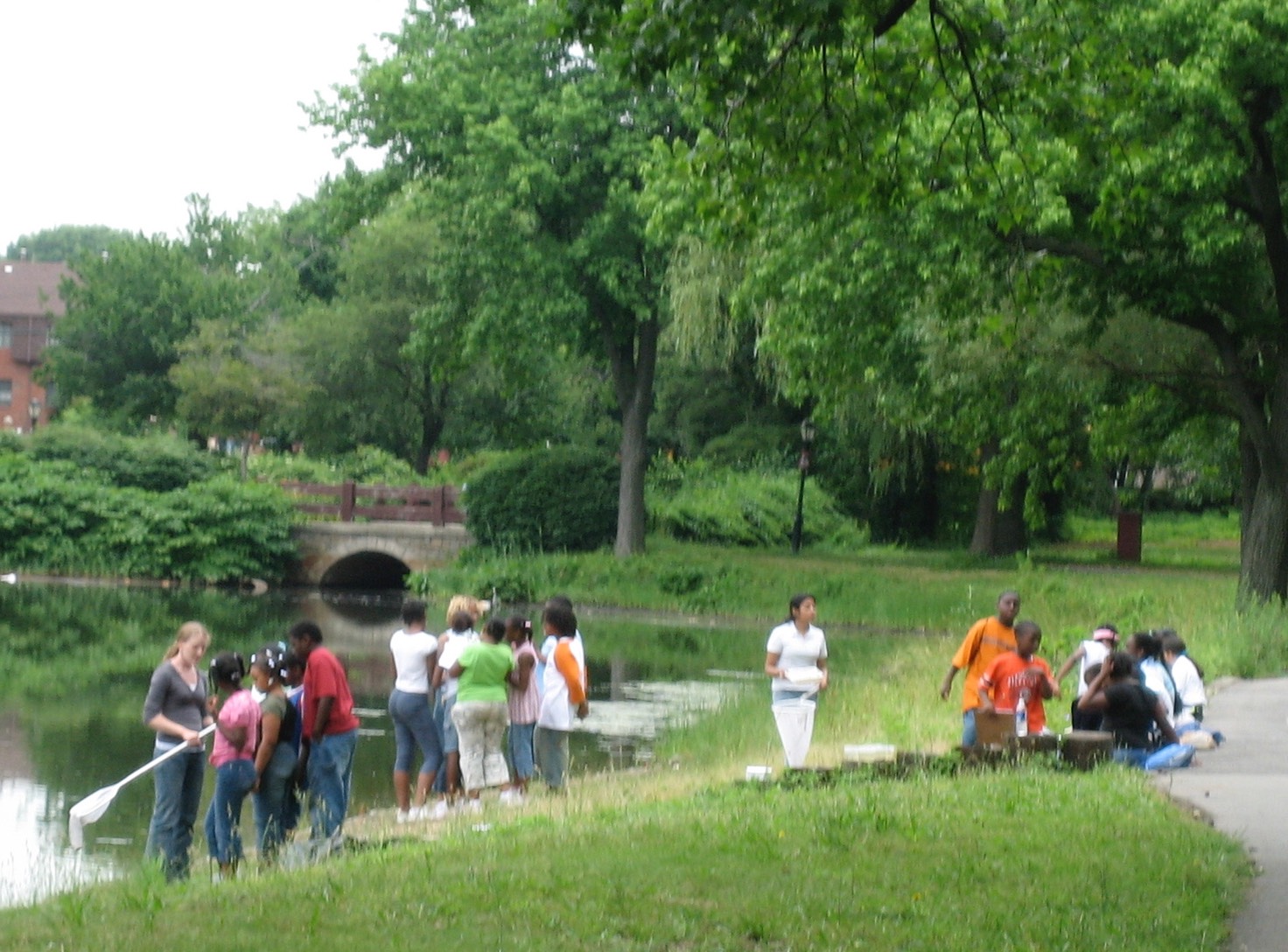This landscape photograph captures a lively scene at a park or a conservation area by a lake. In the foreground, lush green grass leads to a group of children and adults sitting on concrete steps, enjoying a picnic with drinks and food scattered around. Notably, the majority of the children are African American, although there are a few Latinos and white people among them. To the right, by the pond's edge, a lady in a white shirt is instructing a group of African American children, demonstrating rowing techniques with a paddle. One child in an orange shirt faces the camera. Another teacher nearby is holding a net and showing the children something from it, while a third adult with a net and a box is engaged in a similar activity. The clear pond is surrounded by lush, tall green trees and various bushes and plants. In the distance, a small brick building with a visible roof and a bridge with a tunnel beneath it add elements of architectural interest to the verdant backdrop.